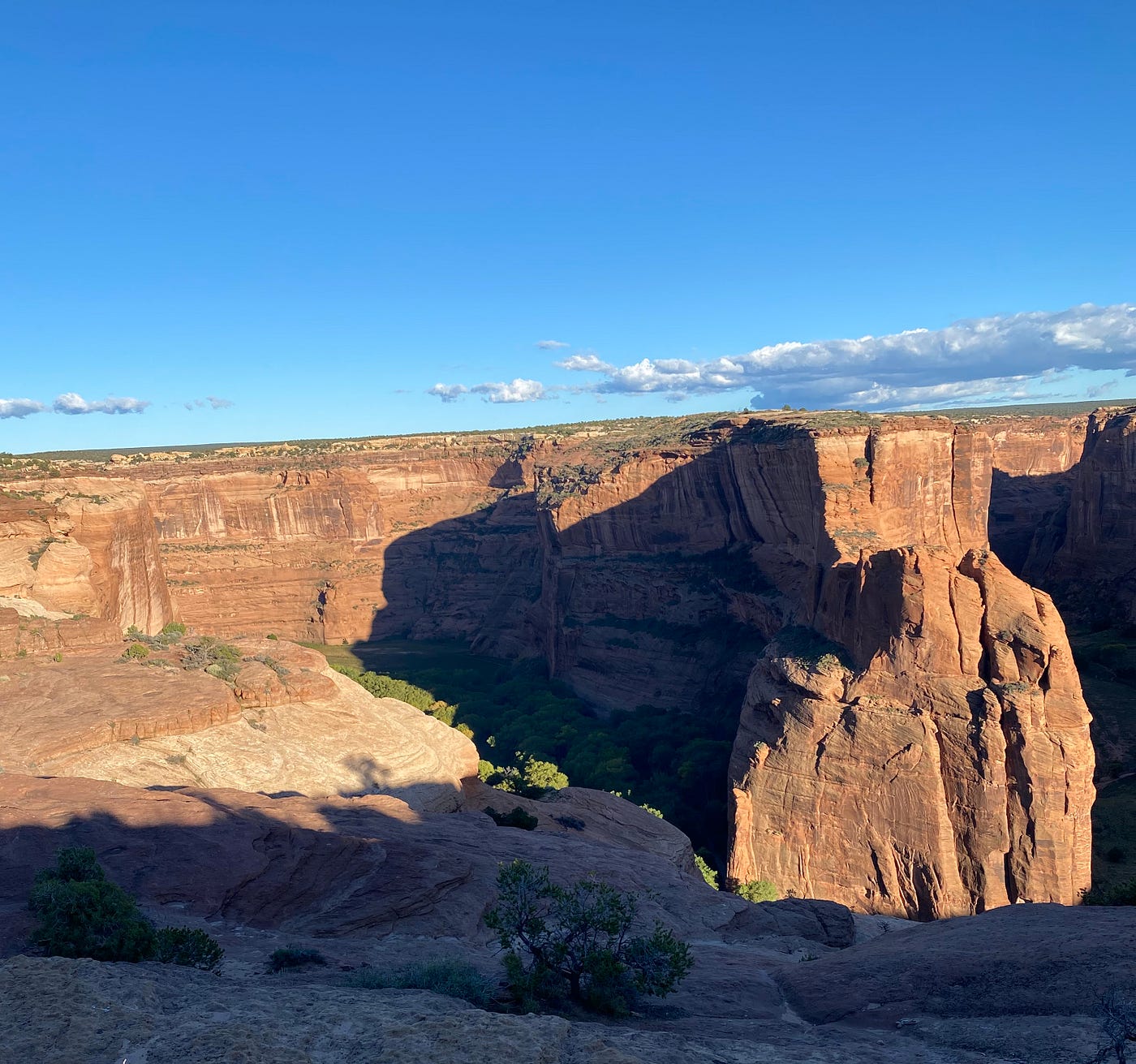The image depicts a majestic canyon landscape taken from a high vantage point during the daytime. The sky above is a vivid blue, dotted with clusters of white clouds, particularly concentrated on the right side of the composition. The canyon itself features striking red and brown rocky surfaces that stretch horizontally from the right to the left side of the image, creating a dramatic visual divide. The base and the surrounding areas of the canyon are adorned with patches of green grass and foliage, with an absence of any human-made structures, suggesting an untouched and natural environment. In the foreground, a cliff edge with green bushes and shadowed areas provides depth to the scene. The ledge appears to drop sharply into the expansive canyon below, adding to the grandeur of the landscape. Despite the canyon's impressive geological formations, there is no river visible, hinting at different erosional processes at play.